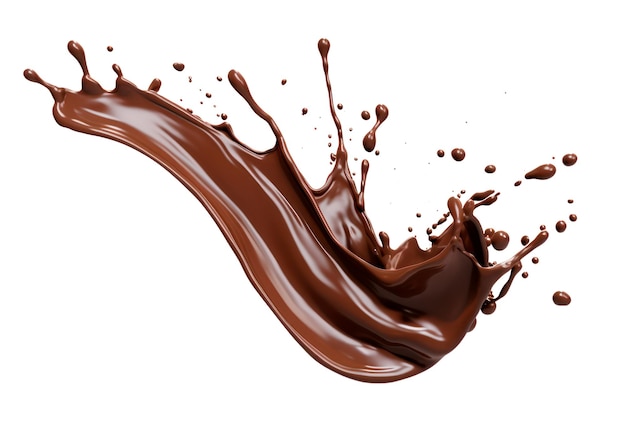The image depicts a dynamic splash of dark chocolate in mid-air, resembling the color and consistency of chocolate pudding. The splash extends from the top left to the bottom middle, curving like a Nike swoosh and creating a thick, slide-like edge closest to the viewer. Numerous smaller droplets cascade off the main splash, adding to its energetic appearance. The background is pure white, highlighting the dark, creamy texture and movement of the chocolate splash, as if it were just thrown into the air.